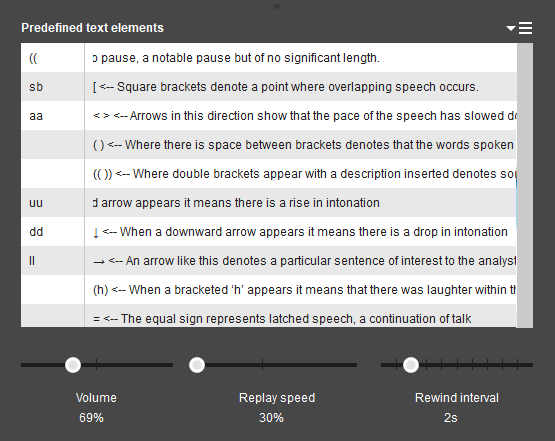This screenshot, taken from a computer screen, showcases a user interface featuring predefined text elements. The interface has a dark gray overall background with an internal section divided vertically. The left section displays a few lines, while the right section, delineated by a vertical line, contains more detailed explanations, featuring longer blocks of text. 

Within the main box, the background alternates between light gray and dark gray in a repetitive pattern. At the top, text elements are categorized, starting with double parentheses "( )". The first entry describes "a notable pause but of no significant length." Following this, "SB" is explained as "square brackets to denote a point where overlapping speech occurs."

Next, "AA" in lowercase letters is accompanied by a note that "arrows in this direction show that the pace of speech was slowed down." Another set of parentheses is mentioned, indicating that "a space between brackets denotes that the word spoken has been cut off." The explanation for double parentheses "(())" begins with "where double brackets appear with a description," but the text is cut off mid-sentence.

Further down, "UU" is defined as "arrows appear, it means there is a rise in intonation." The detailed guidelines and descriptions continue in a similar format all the way to the bottom of the section, where it concludes with a trio of dots, each paired with sliders.